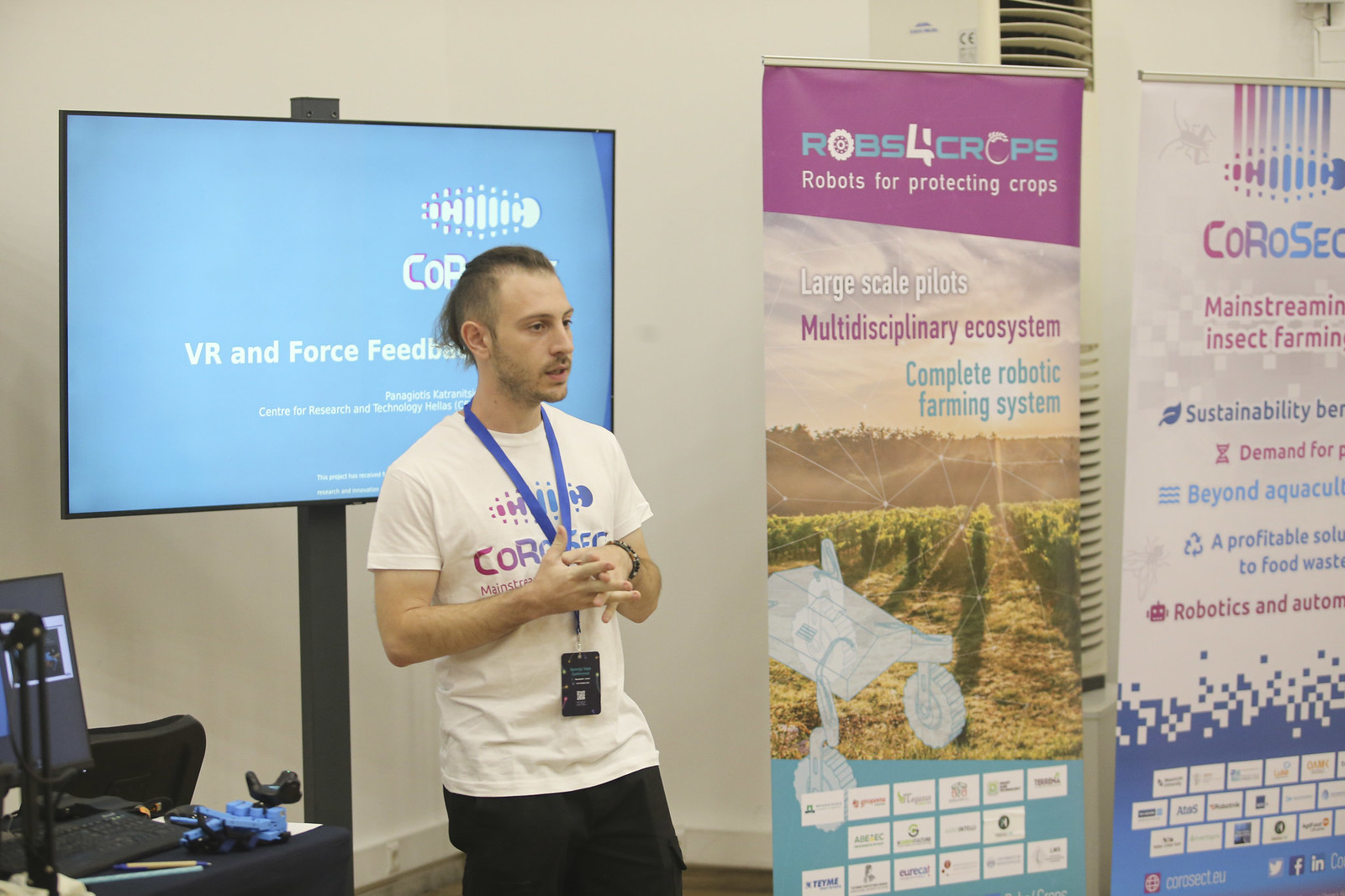The photograph shows a young man, possibly in his 30s or 40s, standing in what appears to be an indoor trade show or convention booth. The man has a high forehead, sideburns, stubble, and is wearing a white t-shirt displaying a partly obscured company logo. He is also sporting a blue lanyard with a black tag and dark pants. His hair is shaved on the sides, and he has his arms crossed in front of him.

In the background, there is a television screen with a blue background displaying the partially obscured text "C-O-R-V-R, Enforced Feedback." The booth showcases multiple posters and banners. One of the prominent posters reads, "Robots for Protecting Crops, Multidisciplinary Ecosystem, Complete Robotic Farming System," indicating a focus on agricultural robotics. Another poster mentions, "Coral Sec Mainstreaming Insect Farming, Sustainability Demand, Beyond Aquaculture, A Profitable Solution for Food Waste, Robotics," though it is partly cut off. The background wall of the booth is gray or off-white with a vent visible in the upper right corner.

Overall, the detailed setting and the man's presentation suggest he is promoting a robotic farming system designed to enhance agricultural efficiency and sustainability.